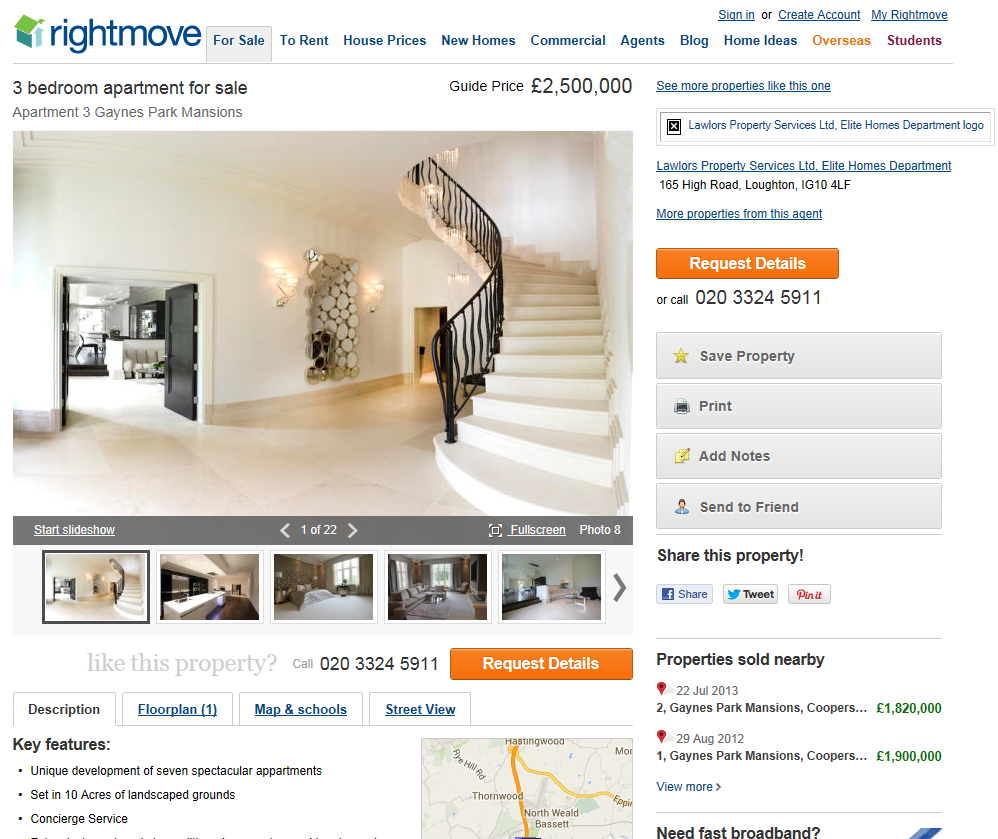**Detailed Caption for Listing Image on Rightmove Website:**

The image is a detailed desktop screenshot of a property listing on the Rightmove website, identifiable by its distinctive house-shaped logo. At the top right corner, users are prompted with options to "Sign in," "Create account," or access "MyRightmove." Below the Rightmove logo, navigation options are displayed, including "For Sale," "To Rent," "House Prices," "New Homes," "Commercial," "Agents," "Blog," "Home Ideas," "Overseas," and "Students."

The current listing in focus is a "Three-Bedroom Apartment for Sale," with a guide price of 2,500 euros. The property is labeled as "Apartment 3, Gaines Park Mansions," and the listing offers 22 images for prospective buyers to view. The image currently highlighted showcases a luxurious curved staircase, indicative of the mansion's opulent interior, featuring ornate mirrors, sophisticated lighting, and elegant tile work.

Users have the option to either start a slideshow, click through images individually, or view the images in full screen. The snapshot is on photo number eight, with the previous images displaying rooms that potentially include a bathroom, bedroom, and living room, with one image that is not clearly identifiable.

Further details provided include a contact number (020-3324-5911) to inquire about the property, and options to "Request Details." Below the main image section, there are categories for "Description," "Floor Plan," "Maps & Schools," and "Street View." Key features highlight the unique development consisting of seven spectacular apartments set in 10 acres of landscaped grounds, complemented by concierge services.

To the right of the listing, there is a section suggesting similar properties and a placeholder image for "Lawlor's Property Services, LTD, Elite Home Department," located at 165 High Road, Loughton, IG104LF. Links allow users to view more properties from this agent, request further details, or call the provided number. Additional interactive options include saving the property, printing the listing, adding notes, sending the listing to family, and sharing via Facebook, Twitter, and Pinterest.

The listing also mentions properties sold nearby, including "Two Gaines Park Mansions, Coopers," sold for 1,820 euros on July 22nd, 2013, and "One Gaines Park Mansions, Coopers," sold for 1,900 euros on August 29th, 2012. There's an invitation to view more similar sales and a brief advertisement about fast broadband services.

In summary, this is a comprehensive listing of a luxurious mansion apartment on the Rightmove website, providing extensive details and user navigation options to facilitate the property search for potential buyers.